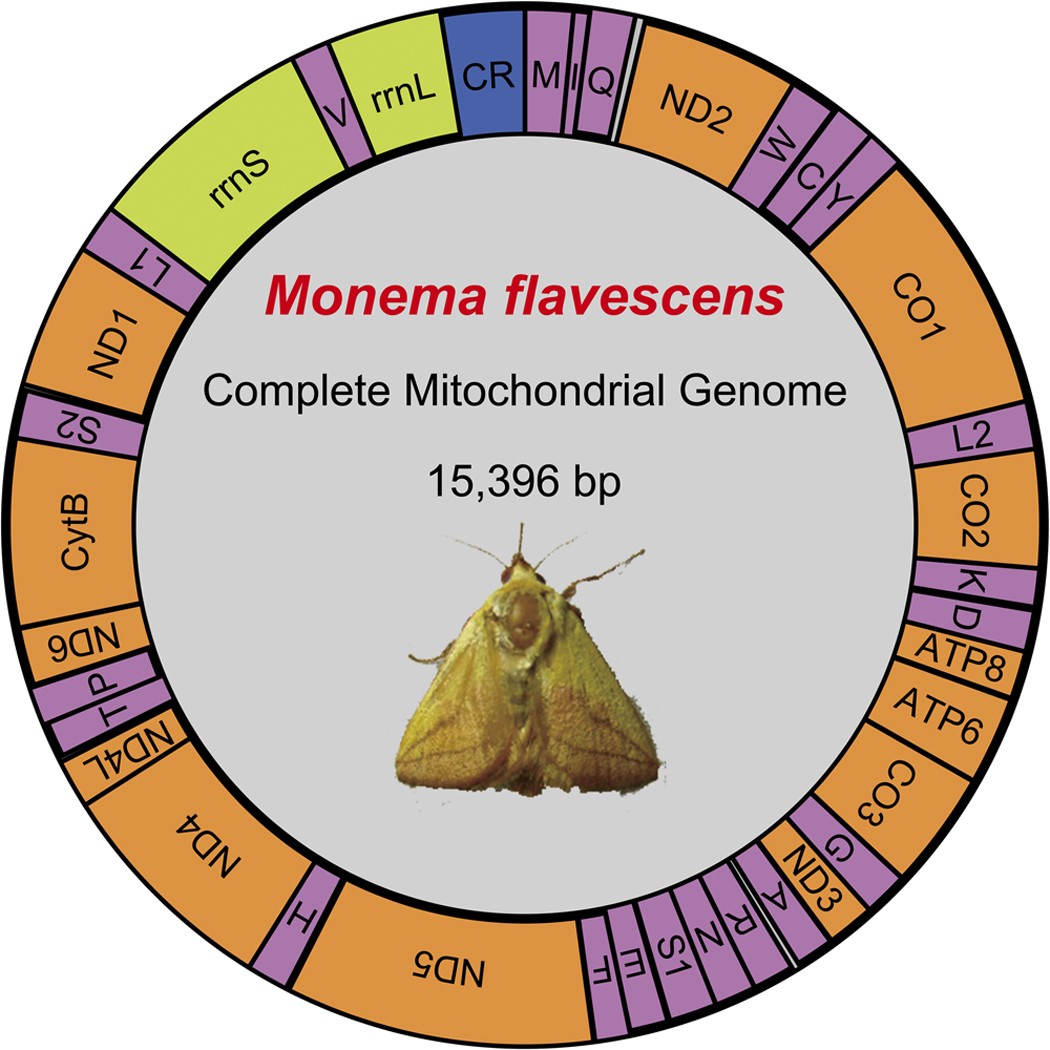The image is a detailed infographic featuring a circular illustration against a white background. At the center of the illustration is a large gray circle with red text at the top reading "Monema Flavacens" and black text below stating "Complete Mitochondrial Genome, 15,396 BP." Below this text is a photograph of a beige, fuzzy-looking moth with discernible antennas and legs, giving the appearance that it is floating atop the gray circle.

Surrounding the gray circle is a segmented wheel chart with various colored sections, each labeled with technical abbreviations such as "RRNS," "RRNL," and "CO1" in black text. The segments vary in width, with the orange sections being the largest, and interspersed with thinner purple, yellow, and a single blue section towards the top. The entire graphic combines elements of photography, illustration, and detailed textual information, presenting a comprehensive visual representation of the moth's complete mitochondrial genome.